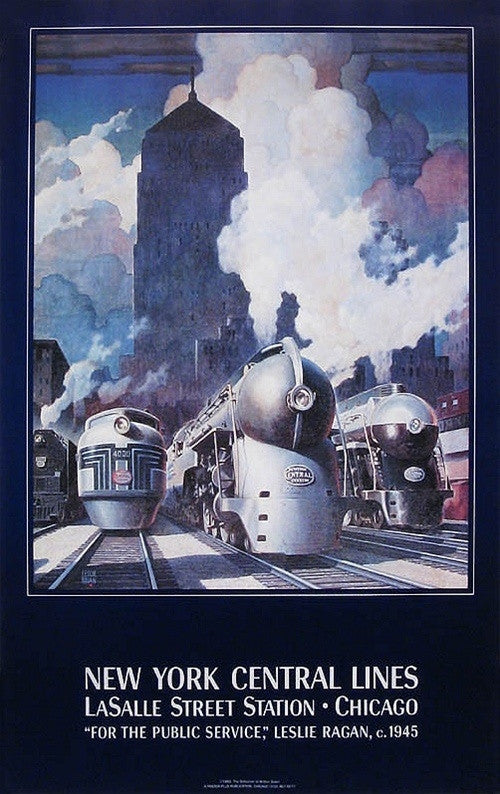The image depicts a vintage 1945 poster for the New York Central Lines, specifically promoting LaSalle Street Station in Chicago. Central to the artwork are three prominently positioned trains, each portrayed with a mix of black and silver tones. The middle train is particularly detailed, displaying a black top with a silver bottom, while the train on the right has a silver top with a black bottom, and the one on the left is predominantly silver. A barely visible fourth train, enveloped in bellowing smoke, can also be seen to the left. This smoke forms cloud-like structures around a background skyscraper, enhancing the depth of the cityscape, which is woven into the smoky sky of blue, grey, and subtle pink hues.

The artistic style reflects a futuristic vision from 1945, capturing the grandeur of railway transport with an evocative sense of motion and industrial strength. There are faint traces of human figures on the middle train, but they remain indistinct against the overall bustling scene. The tracks beneath the trains are clear, leading directly toward the viewer, creating a dynamic perspective.

This detailed artwork is bordered by a thin white outline and encased in a black frame. Beneath the image, white text on the black background reads: "New York Central Lines, LaSalle Street Station, Chicago, for the public service, Leslie Ragan, copyright 1945," with further fine print text at the bottom center that is difficult to discern. The overall composition seamlessly combines the elements of steam, architecture, and motion, celebrating the era's vision of railroad progress.